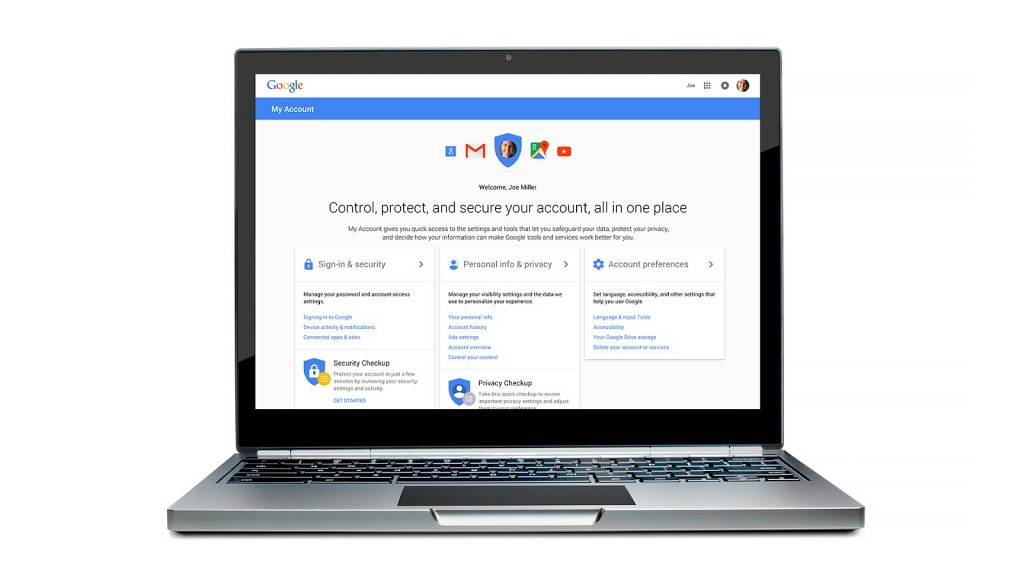This image features an open laptop with a grey keyboard area. The trackpad and keys are black, as is the border around the screen. A circle in the middle of the border is the laptop's camera. The laptop is displayed on a transparent background.

The screen of the laptop is open to a Google account page. In the top left corner, the Google logo is prominently displayed, and beneath it spans a blue banner with "My Account" written in small letters on the left side. In the top right corner of the screen, there are four icons, with the fourth being an avatar photo of the account holder.

Centrally, the page greets the user with a welcome message followed by the user's name. Below this, it displays the text: "Control, Protect, and Secure Your Account, all in one place" in black letters. Just above this message are five logos representing Google services: Mail, the Security Centre, Google Maps, and YouTube.

At the bottom of the page are three distinct boxes. The first box, on the left, is titled "Sign in and Security," the second box is "Personal Info and Privacy," and the third is "Account Preferences," each containing descriptive text outlining their functions.